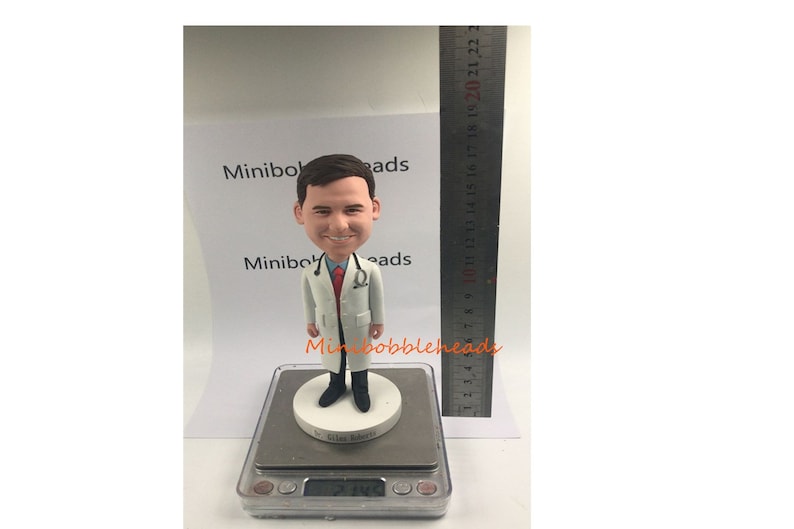This image depicts a highly detailed mini bobblehead figure of a doctor standing on a small, grayish scale. The doctor, who has white skin and dark brown hair, is wearing a white lab coat over a blue polo shirt and a red tie, paired with black pants and black shoes. A stethoscope hangs around his neck, completing his medical appearance. The bobblehead stands on a white circular pedestal akin to a coaster and is marked at the bottom with the name "Dr. Giles Roberts," though the text is quite small and partially illegible. The scale displays the number "2145," although the weight cannot be clearly discerned. A silver ruler positioned to the right of the figure indicates its height, approximately 17 to 18 centimeters. Behind the bobblehead, a sheet of printer paper reads "mini bobbleheads" twice, albeit partially cut off. The same phrase, "mini bobbleheads," is written in orange, cursive font across the front of the image, possibly for copyright protection. The doctor is smiling cheerfully, adding a touch of charisma to the figurine.